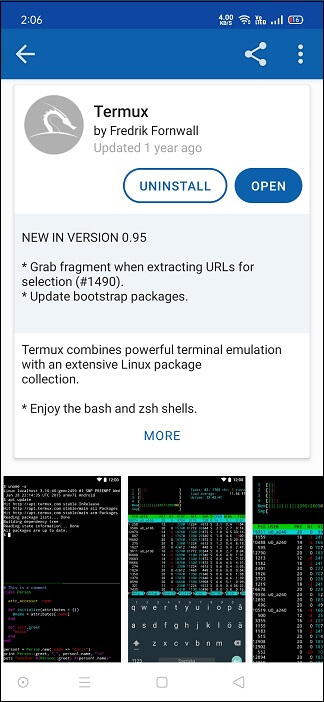Screenshot of the Termux app's listing in an app store, possibly the Google Play Store. The app, developed by Frederick Thornwall, was last updated one year ago. At the top of the screen, "Termux" is prominently displayed, with the developer's name immediately below it. To the right, there are two buttons: a white "Uninstall" button and a blue "Open" button. Further details reveal the latest update (version 0.95), which includes a new feature for grabbing fragments when extracting URLs for selection (noted as issue #1490), and an update to bootstrap packages. Termux is described as a combination of powerful terminal emulation and an extensive Linux package collection.